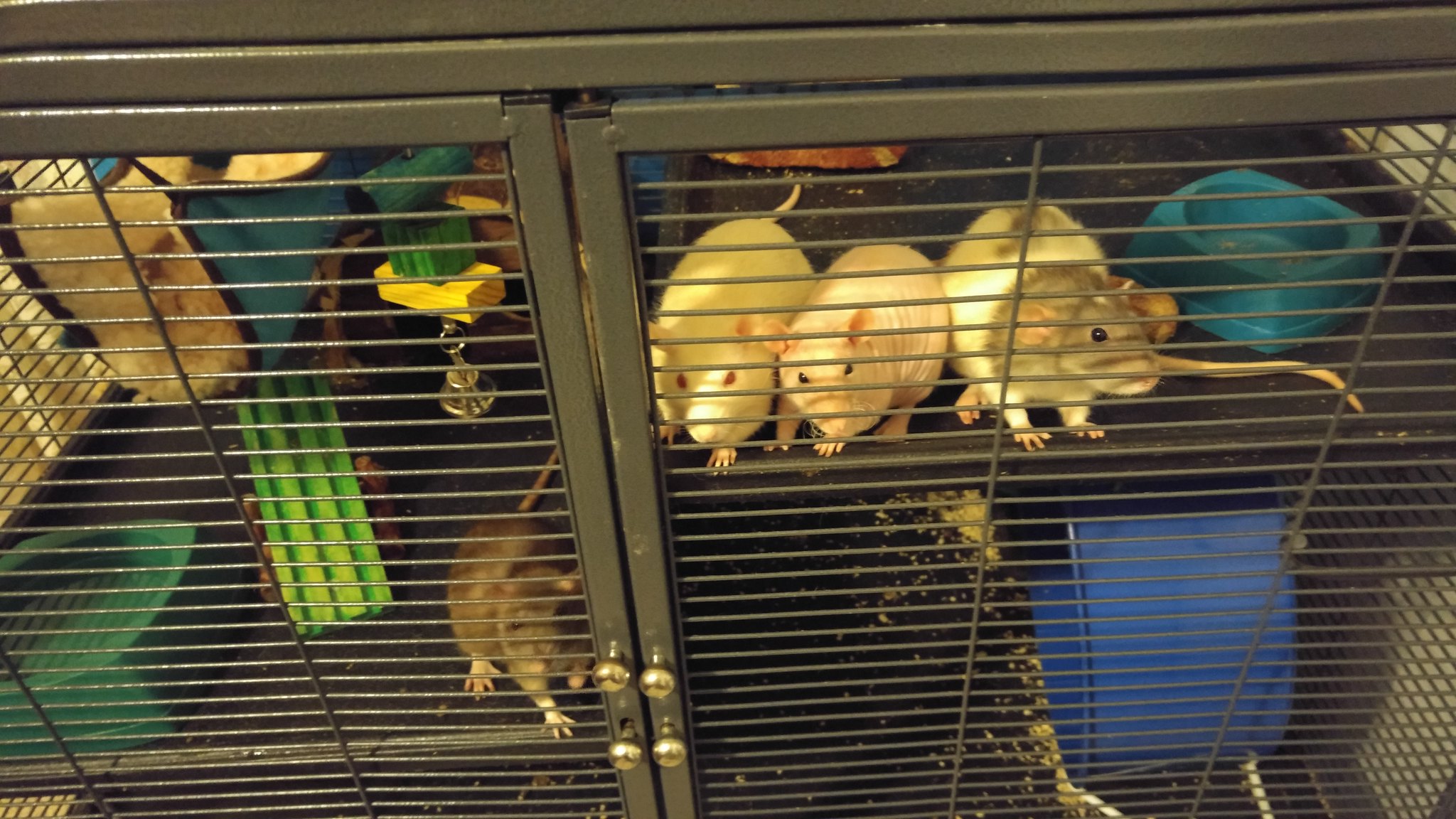This image, likely taken in a pet store or by a rat enthusiast, is a detailed look into a spacious, powder-coated brown metal cage with multiple levels. The cage, viewed from a slight diagonal angle, features double doors at the front, each adorned with a pair of brass knobs—one set at the top and another at the bottom. Inside, on an upper-right shelf, three small rodents are visible: an albino mouse with red eyes, a hairless pink mouse with black eyes, and a white and gray mouse with dark eyes. These animals are near a turquoise plastic feeding bowl containing some crumbs. Beneath this shelf, the image reveals a vertical exercise wheel surrounded by scattered pine shavings. On the left side of the cage, another shelf holds various chew toys made of colored wood, a small bell, and a green bowl. Nearby, a brown rat, with its paw touching the wire bars, adds to the lively scene. In the background, a chunk of cedar or another chewable item is visible, contributing to the enriched environment for these small pets.